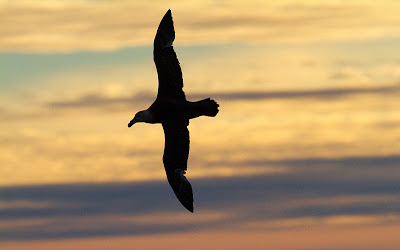This artistic photograph captures a silhouette of a seagull in flight, its wings spread vertically as it glides leftward across the scene. The seagull stands out in sharp contrast due to the strong backlighting, making the bird appear as a striking black silhouette. The background features a soft, out-of-focus beach or ocean with waves subtly visible at the bottom of the frame. The sky transitions through a gradient of colors, from muted pinks and purples to oranges and blues, indicative of a sunset or sunrise. Stratus clouds occupy the top quarter of the image, with a small strip of clear blue sky peeking through, adding depth and visual interest. The overall composition, with its focus on the seagull and the harmonious interplay of colors, presents a serene and visually captivating scene, suitable for framing and display as a piece of art.